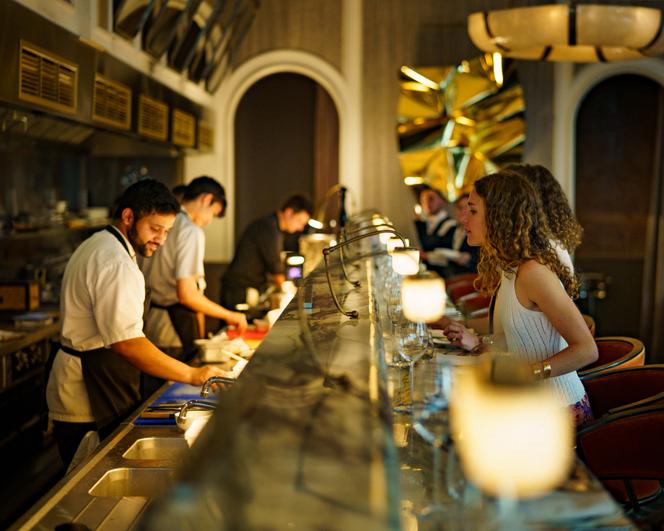In this digital photograph, a woman with frilly hair, dressed in a sleeveless white tank top, is seated at a cozy cocktail bar, illuminated by warm yellow lights above each patron. She appears to be contemplating her order while attentively watching the friendly and down-to-earth bartenders preparing drinks. Surrounding her are various patrons, who seem less approachable. The bar is stylishly equipped with glass lamps, tables, chairs, and eating utensils. This vibrant scene is primarily adorned with shades of brown and white, but also features touches of blue, gold, red, and green, adding to its inviting atmosphere. The right side of the image showcases people being served at a buffet-style countertop, with three staff members actively preparing food.